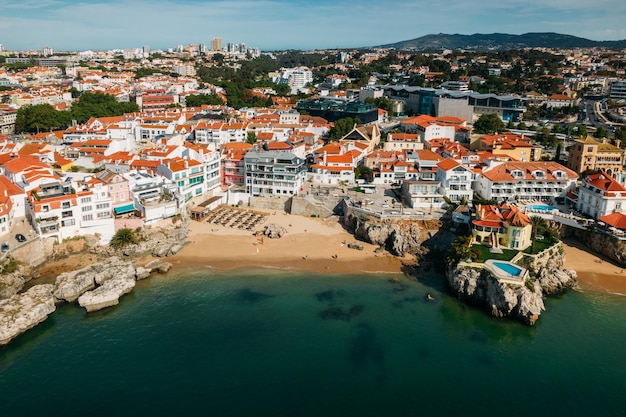This horizontal aerial view captures a picturesque beach scene with a blend of natural and architectural elements. The foreground features a clear, bluish-green body of water juxtaposed with the sandy beach dotted with large, silver-gray rocks. The beach lies towards the bottom left and middle of the image. Nestled along this beach are numerous buildings, likely hotels or resorts, distinguished by their reddish, brownish-orange roofs. One prominent building to the right sits slightly elevated on a small island, fronted by a swimming pool. In the background, a series of mountains rise under a blue, cloudy sky, adding depth to the scene. Despite the image being slightly blurry, the composition effectively showcases a serene coastal landscape with the interplay of beach, water, rocky elements, and the distant mountains.